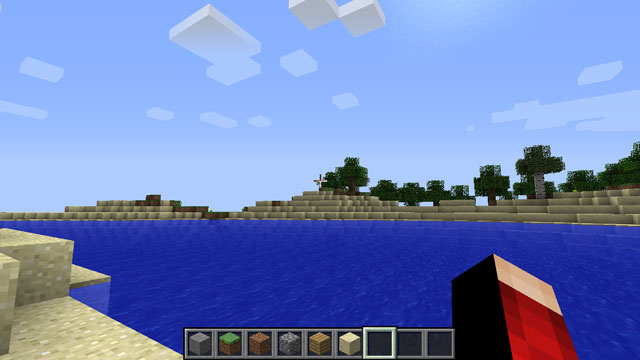This screenshot captures a digital artwork tool interface, possibly used for designing virtual environments. Dominating the image is a central body of translucent water flanked by cement brick barriers on each side, reflecting a meticulous attention to detail. Above this tranquil water, the background showcases crudely drawn green trees under a light blue sky, which intriguingly features floating squares acting as clouds. In the foreground, an interface element presents a variety of brick texture options: from gray to brown with a green top, plain brown, cobbled gray, lighter brown, to a matte light gray. Below these textures, three horizontal blank boxes are available for selection. Adding an element of intrigue, a large red brick juts out over the water, its end shaded gray and one side black, contributing to the surreal and imaginative aesthetic of the scene.